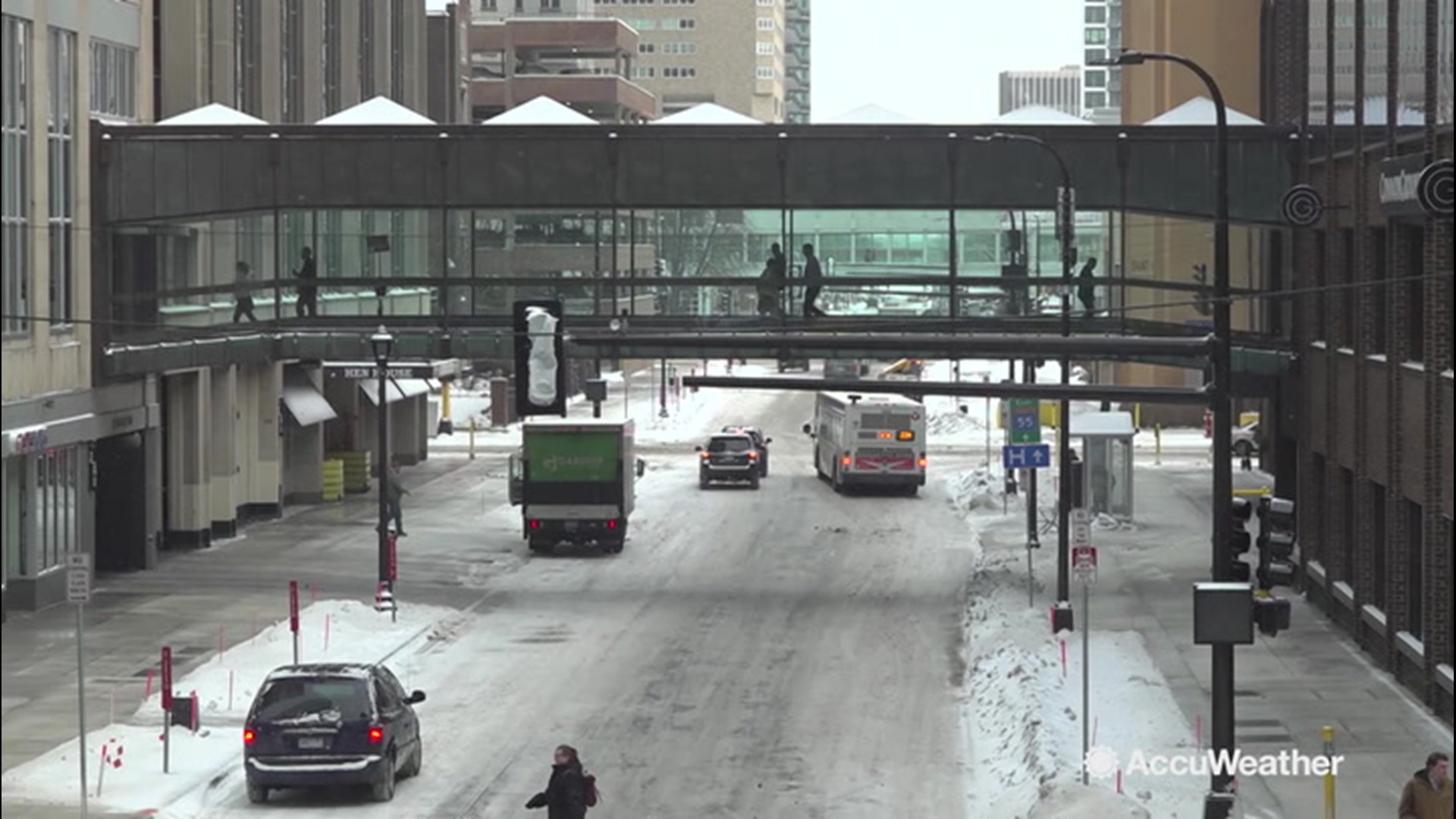The image captures a bustling downtown urban street, likely in Minneapolis, Minnesota, on a cold winter day. The centerpiece is a black Skyway walking bridge adorned with patches of snow, stretching horizontally from left to right. The bridge links a multi-storied building with a lighter gray facade on the left to a glass-paneled high-rise on the right. There are at least four people walking inside the bridge. 

Below the Skyway, at street level, a lady wearing a black jacket can be seen crossing the icy, snow-packed road, where several cars and a blue bus are driving cautiously. To the left of the street, near the curb, parking meters peek out from the snow, alongside a parked car with its taillights illuminated and a green and white delivery truck.

The sidewalks, cleared of snow, are dotted with street signs and a red bus stop sign. A blue hospital direction sign with an arrow points towards an unseen location. The bustling scene is complemented by traffic lights and a light post starting in the lower right-hand corner of the image. In the background, several buildings rise against the overcast, cloudy sky, contributing to the mood of a frigid winter's day. Overlaying the bottom portion of the right side is the AccuWeather logo, featuring a sun icon, marking the image with a recognizable weather brand.